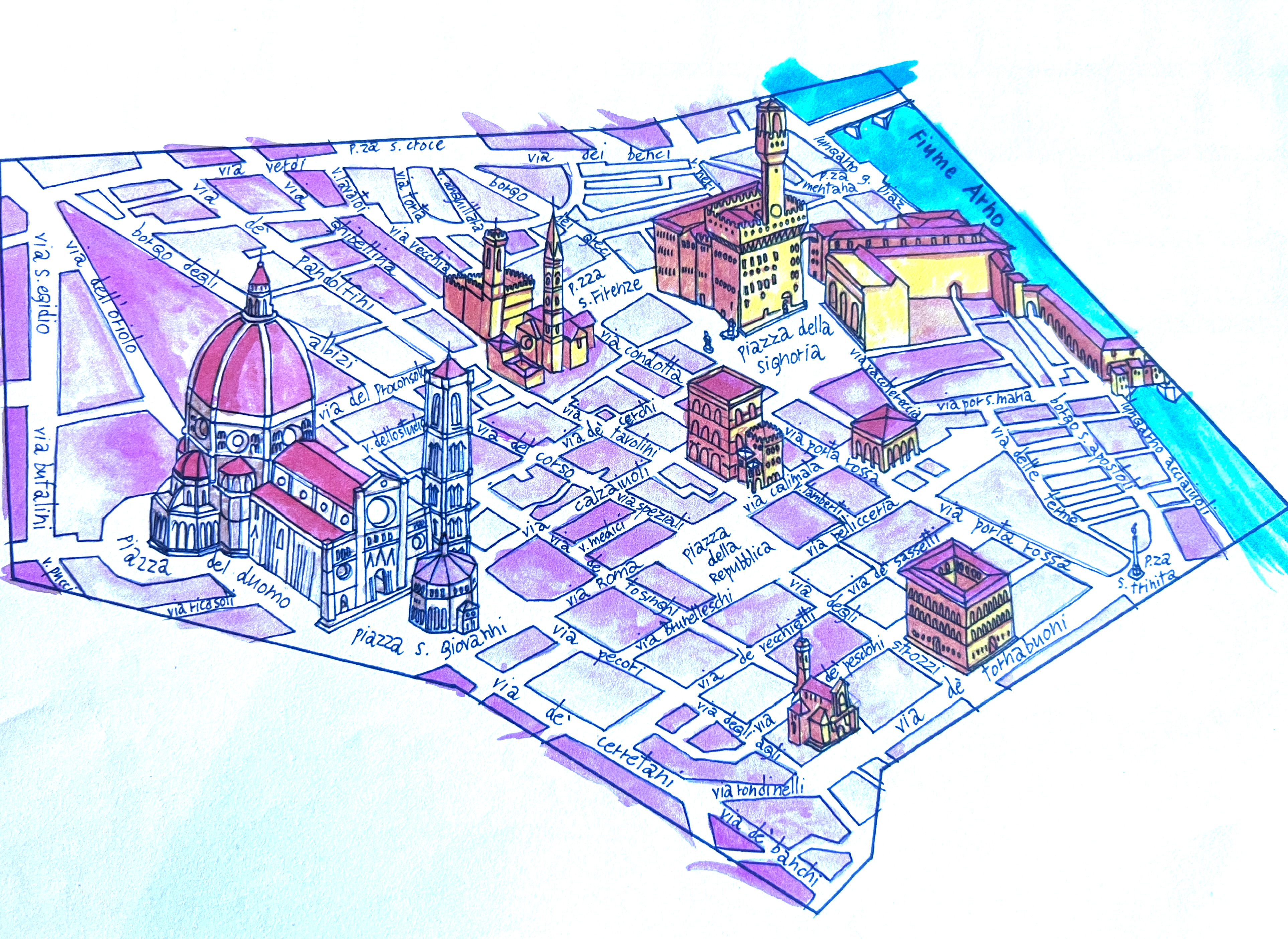This hand-drawn, 3D-like map of an Italian city is rendered with a mixture of watercolor and blue pen. The map features labeled streets and landmarks in Italian, creating an intricate and detailed representation. Prominently, historic buildings such as those in Piazza del Duomo, Piazza del Giovanni, and Piazza della Signoria are superimposed on the map, sticking up to give a three-dimensional feel. Many of these buildings are illustrated with plum or purple hues, with white highlights indicating lighting, while some structures also boast yellow walls and red roofs. On the far right, the Fiume Arno flows, with bridges arching across the river. The background is a soft blend of light blue and white, while the spaces between the streets and buildings are filled with a purple color, demarcating plots of land. This picturesque map skillfully combines detailed architectural illustrations and vibrant colors to convey a vivid glimpse of an Italian city's layout.